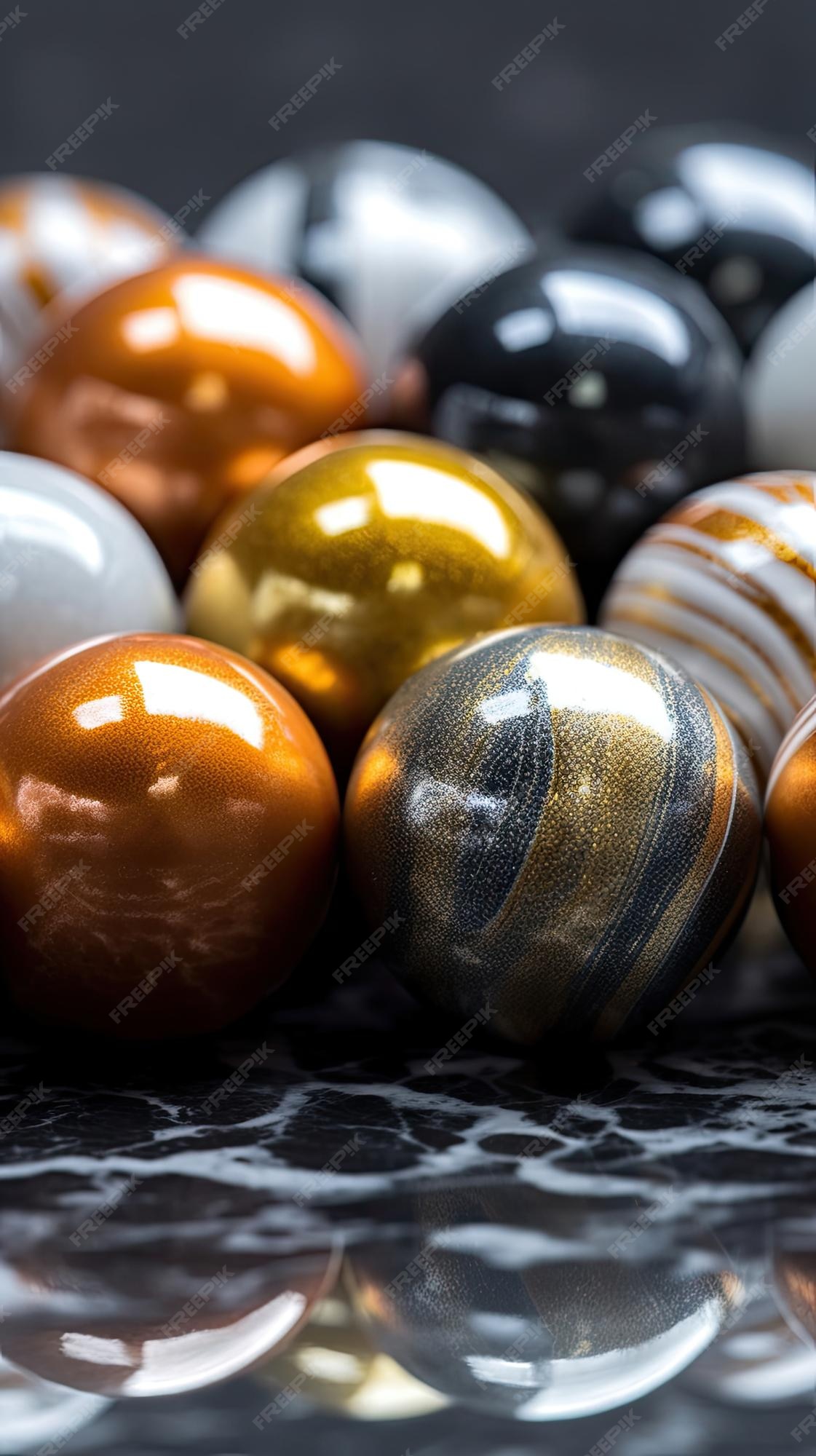This image captures an exceedingly close-up view of twelve shiny orbs resembling marbles or beads, arranged on a black marble surface intricately veined with white and gray. The marbles vary in appearance, featuring both solid and multi-colored designs. Predominantly, the marbles exhibit bold, lustrous hues—solid colors like bright gold, vibrant orange, stark black, and pristine white stand out vividly. 

Further adding to the visual interest, some marbles are intricately swirled with colors reminiscent of planetary rings, evoking the sights of Jupiter or Saturn; these swirled marbles are adorned with multiple layers of blue, gold, and brown. One particularly striking marble in the center is entirely golden, drawing the eye. Other notable marbles include those with shimmering touches, perhaps giving an illusion of glitter, and marbles with alternating stripes of gold, black, and white.

Despite differing materials that make it difficult to discern whether they are metallic or glass, the marbles’ polished surfaces reflect light to create a radiant, glossy effect. The detailed textures and contrasting colors set against the elegant marble background lend a realistic and visually compelling quality to the image.